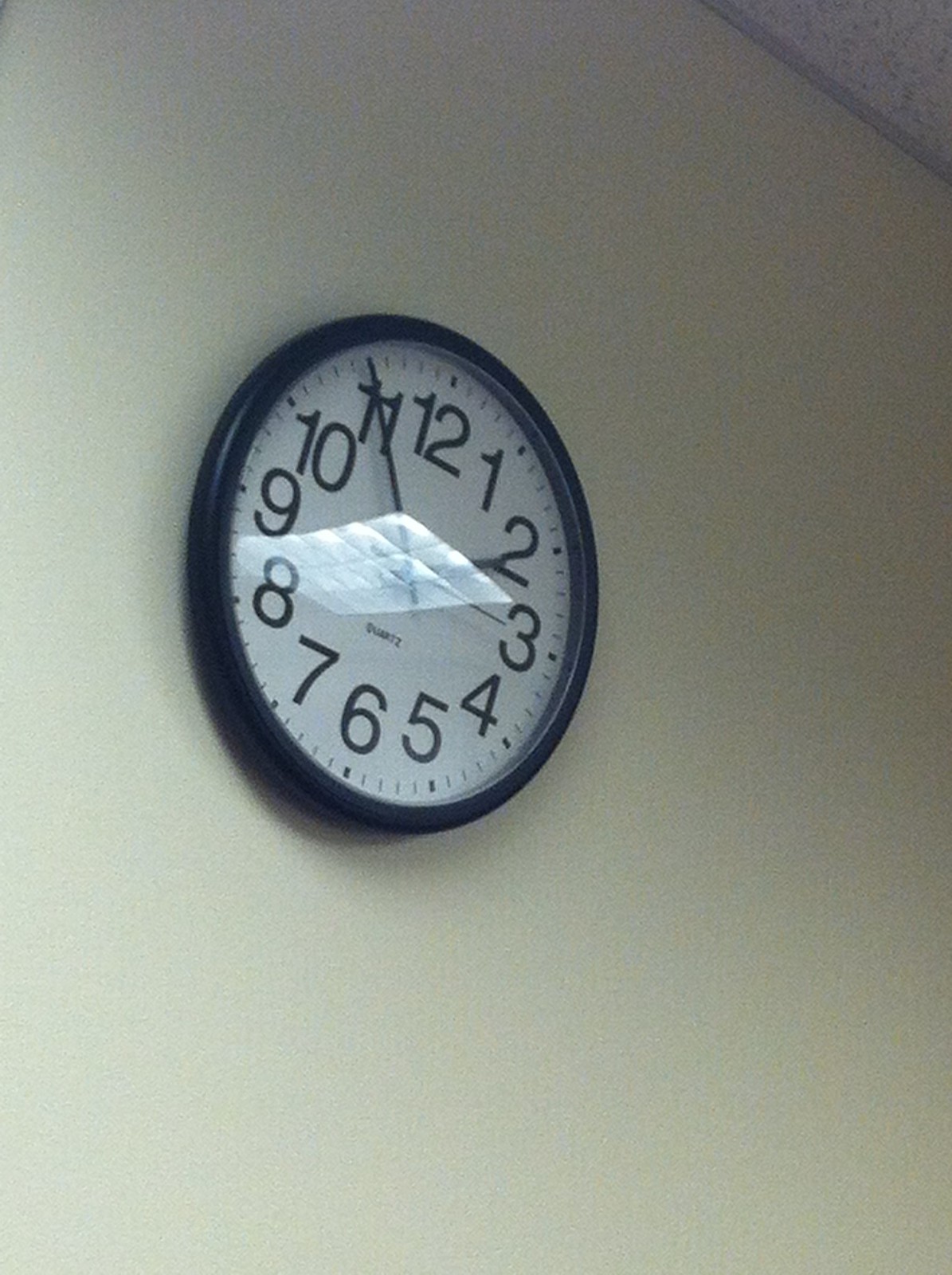The photo features a classic black-bordered wall clock, typical of those found in schools. The clock face is bright white with large black numbers marking the hours and smaller marks indicating the minutes, with more pronounced marks for the five-minute intervals. The hour hand is positioned at the 2, the minute hand at the 11, and the red second hand at the 3, displaying a time of approximately 1:55. The word "Quartz" appears in black at the center of the clock. The clock is mounted on a wall with a light tan color, which appears slightly shadowed. The image is taken in portrait mode from a slight angle to the left, creating a noticeable glare on the clock face. Part of the ceiling is visible at the top right corner, enhancing the perspective of looking up at the clock.